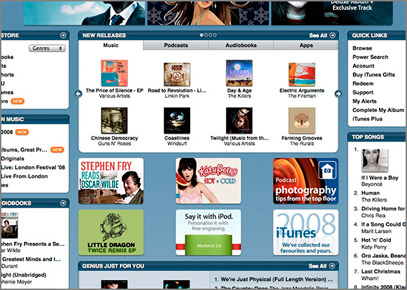The image features a vibrant blue background. At the very top, there are partial views of three images. The first image shows a clear blue sky with white clouds and a man wearing a dark suit, white shirt, and tie. The second image portrays a woman with exceptionally long hair. The third image is labeled "Exclusive Track."

On the left side, there are three boxes, each displaying a dark blue top and a white bottom. Some of these boxes are marked with red "NEW" labels. Central to the image is a section titled "New Releases" on a dark blue background. This section includes four circles: the first one is white and labeled "See All," followed by categories such as Music, Podcasts, Audiobooks, and Apps. Below this title, there are eight items available for selection, bordered by a small white left arrow on the left and a white right arrow on the right.

Additionally, the middle row shows six more covers, with a prominent green button located in the center image at the bottom. The top of this section also features a dark blue banner reading "Just For You" alongside a "See All" option. Here, more images are displayed.

On the right side of the image, under a dark blue "Quick Links" banner, is a section listing options like Browse and Power Search against a white background. Below this, there is another box: it has a blue top with the title "Songs" and a white background listing tracks from one to eight, starting with "If I Were a Boy" by Beyoncé.